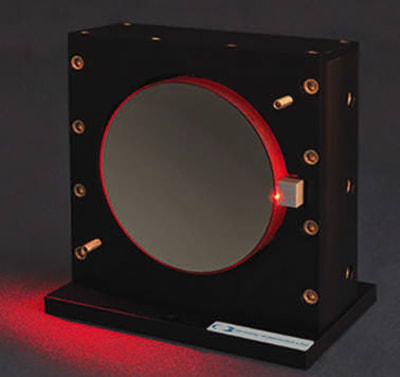This image features a black rectangular structure with a black base that extends slightly beyond the main body. The base sits on a red-illuminated ground, enhancing the visual contrast. Prominently, the structure has rivets along the top, sides, and particularly on each corner, contributing to its industrial appearance. In the center of the structure, there is a gray circular feature bordered by a maroon or red ring, which gives the impression of a mirror or perhaps an illuminated display. To the right of this central circle, a small gray square device with a red LED light is visible, adding to the intricate details of the design. The overall aesthetic suggests a high-contrast graphic art image with elements that evoke a blend of modern technology and classic industrial design.